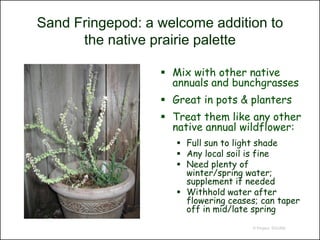The image is an advertisement for a plant called Sand Fringe Pod, designed to appeal to those creating a native prairie palette. The plant, housed in an off-white or gray planter, features green foliage with white flowers and has fewer branches than typical plants. It is set against a background of light wooden fencing, suggesting an outdoor setting. The pot rests on a bed of gray rocks. Key features of the plant are listed in green text on the right side of the ad, including care instructions that recommend mixing with other native annuals and bunch grasses, suitability for pots and planters, and guidelines for watering and sun exposure. The accompanying text emphasizes its compatibility with various soil types and its need for full sun to light shade.